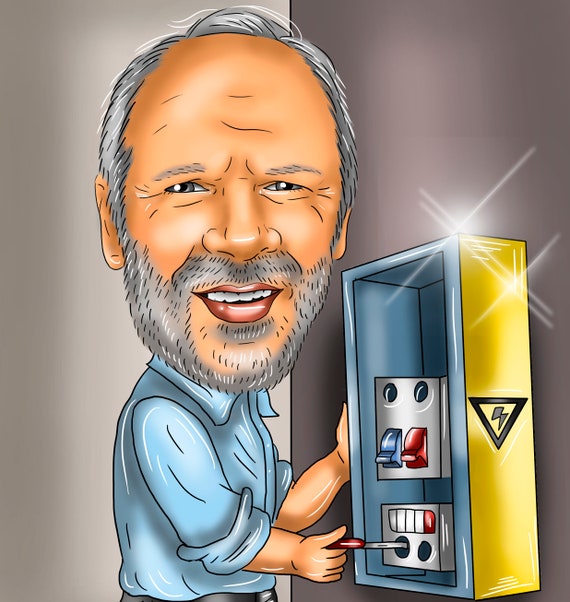This is a detailed digital cartoon drawing of an older white man with gray hair, a neatly trimmed beard and mustache, and a large head typical of caricature art. He has a cheerful semi-smile and squinting eyes, suggesting a friendly demeanor. His attire includes a light blue shirt with rolled-up sleeves and a visible black belt, though only his upper body is shown. He stands facing forward with a screwdriver in hand, seemingly in the process of fixing or adjusting elements inside an open electrical panel. The panel, which features a yellow casing marked with an energy symbol, contains two prominent switches—one blue and one red—and several buttons or components below them. The man appears to be manipulating a twist-lock component that resembles piano keys. The background is a muted gray, providing a neutral backdrop that makes the bright, sparkly lines and vibrant colors of the illustration—predominantly gray, yellow, blue, and red—stand out. This image likely serves as a playful, eye-catching representation for an electrician's website or professional profile.